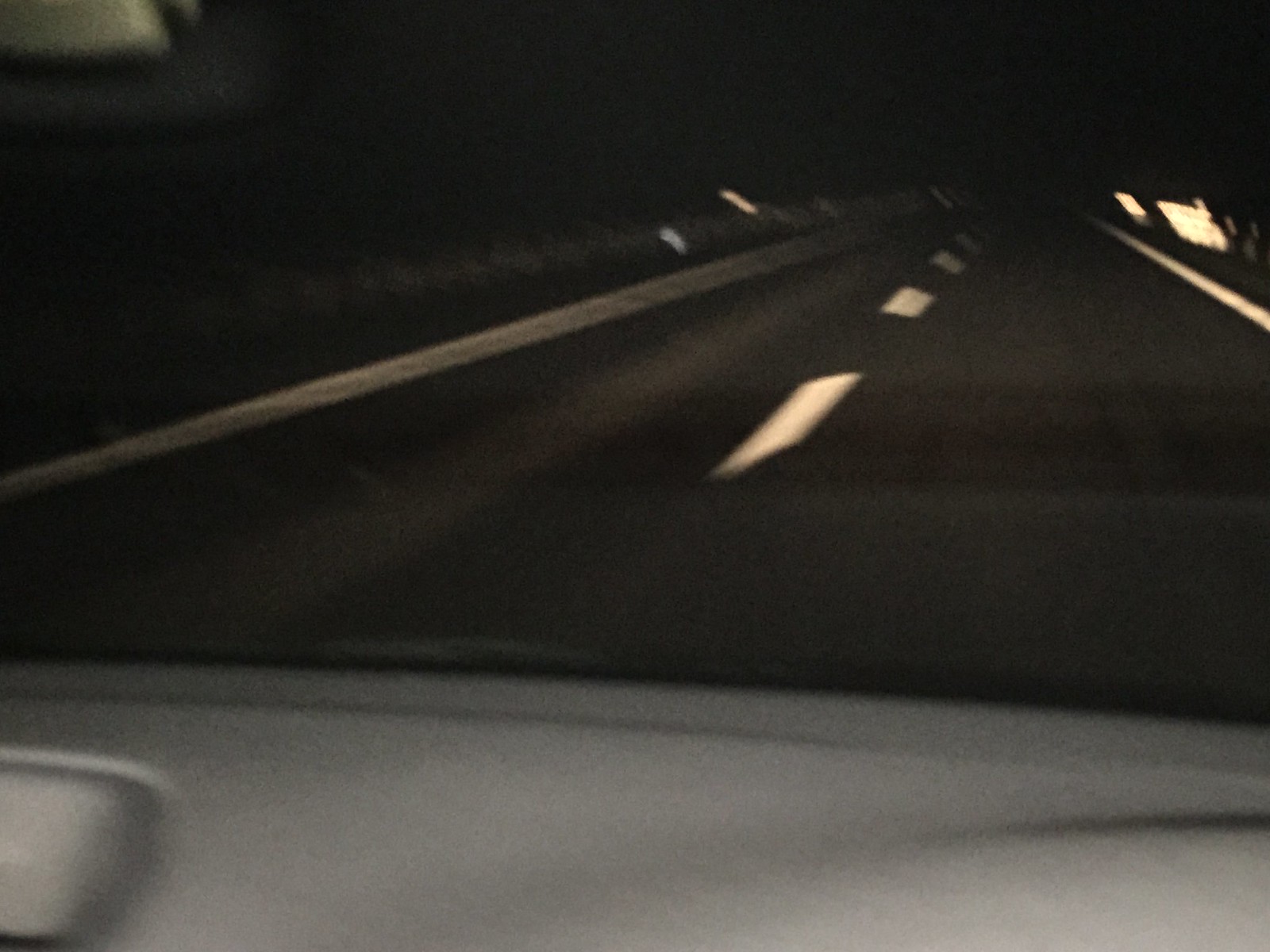A nighttime photograph taken from inside a vehicle showcases a gray plastic dashboard with a visible indent on the left side. Peering through the windshield, a black asphalt road stretches ahead, distinguished by white-painted dashed lines marking the lane. On the right side of the road, two rectangular lights stand out, casting illumination over the asphalt. Further down, another light can be seen on the opposite side, delineating the road’s edges, which are bordered by white lines. To the far left, dust, dirt, and patches of dry grass are noticeable. The sky above is pitch black, offering no visible detail or stars. Positioned at the top left of the image, a rear-view mirror hangs, completing the scene of a quiet, deserted road at night.